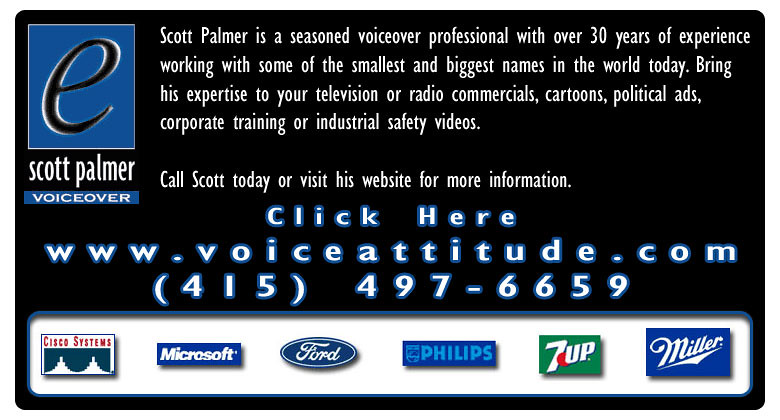The image is a horizontally-aligned rectangular screenshot of a web page promoting voiceover artist Scott Palmer. Dominating the upper left-hand corner is a notable logo, a blue square outlined in white featuring a lowercase 'e' inside. Directly beneath the logo, bold white text states "Scott Palmer," with "voiceover" positioned underneath against a blue background. Centrally aligned, white text describes Scott Palmer as a seasoned voiceover professional with over 30 years of experience, highlighting his versatility in working with a range of clients from small to large. The text elaborates on his expertise, which spans television and radio commercials, cartoons, political ads, corporate training, and industrial safety videos. Below this, readers are encouraged to get in touch with Scott via a call or by visiting his website for more information. Prominently displayed in highlighted white letters with blue outlines is an actionable link reading "click here," followed by the URL "www.voiceattitude.com" and the phone number "415-497-6659." At the bottom of the image, a white rectangular strip outlined in blue lists notable companies from left to right: Cisco Systems, Microsoft, Ford, Philips, 7-Up, and Miller, suggesting they are past clients or sponsors. The background of the entire page is in black, creating a sharp contrast with the white and blue elements.